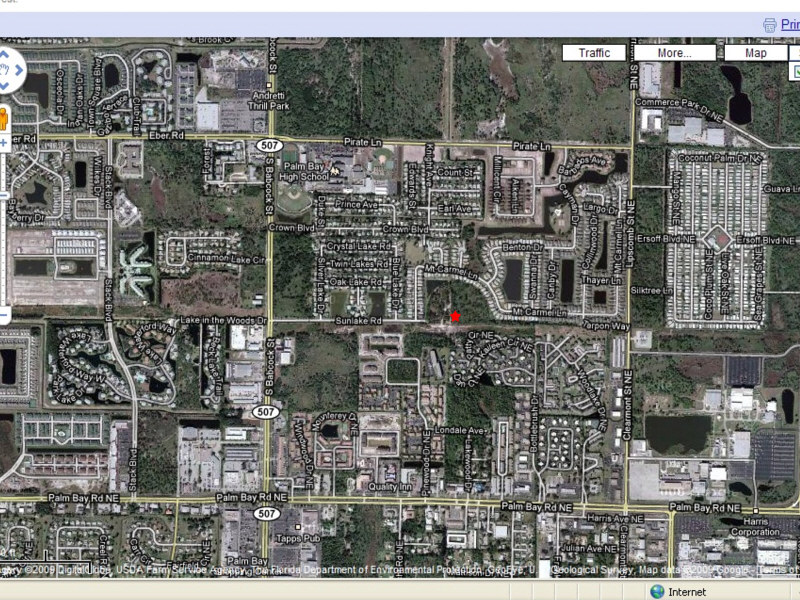This image appears to be a screenshot of a Google Maps interface from 2009, as indicated by the copyright information in the lower left corner. The map also bears fine print crediting the "Florida Department of Environmental Protection Geological Survey" for some of the data. On the left side of the image, you can see the zoom control slider for adjusting the map's scale vertically. In the upper right corner, there are toggle options including white rectangular buttons for "Traffic" and other map features.

The central area of the map showcases a red star marker, which presumably highlights a specific location. Surrounding this focal point are various street names, including Sunlake Road, Mount Carmel Road, Circle Northeast, Count Street, and Earl Avenue. The red star is situated near the main thoroughfare, South Babcock Street, which is designated as Route 507.